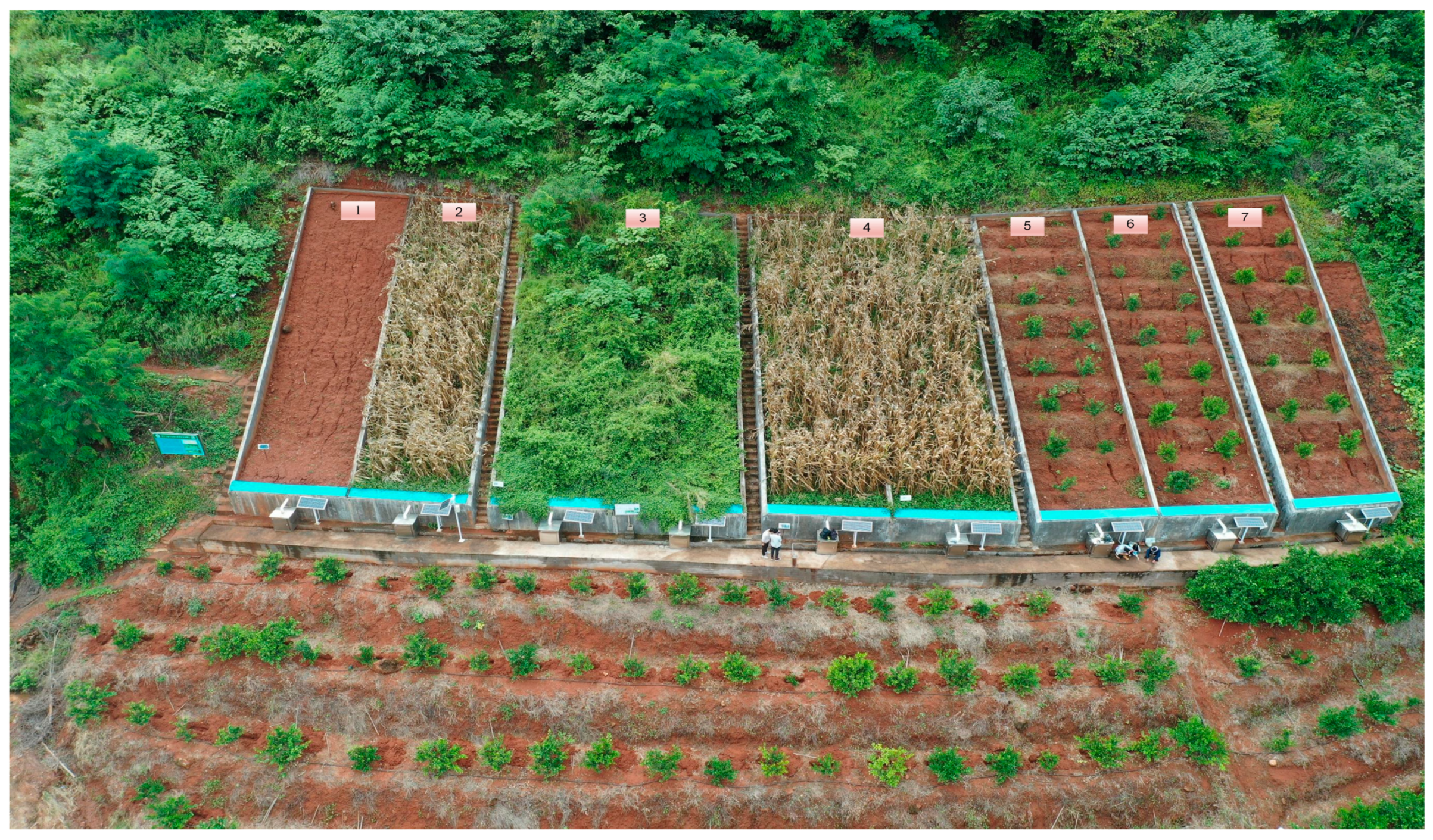This overhead, aerial view captures a sizable garden area segmented into seven numbered rectangles, each showcasing different stages and types of growth. Rectangle 1 appears to be mostly dirt, possibly ready for planting. Rectangle 2 is covered with tan-colored weeds, starting from the bottom. Rectangle 3 is filled with dense green growth, while Rectangle 4 contains a mix of green and tan vegetation. Rectangles 5, 6, and 7 feature organized rows of small green bushes emerging from the brown dirt. In front of these rectangles, a walkway is visible, where several people can be seen, emphasizing the distant perspective of the photograph. Beyond the walkway are three long rows that extend across all seven blocks, featuring mounds of dirt each topped with green bushes similar to those in Rectangles 5, 6, and 7. The scene is framed by lush greenery at the top of the image, contrasting with the neatly organized planting area at the bottom. The overall layout suggests a well-planned yet varied agricultural space, possibly captured by a drone.